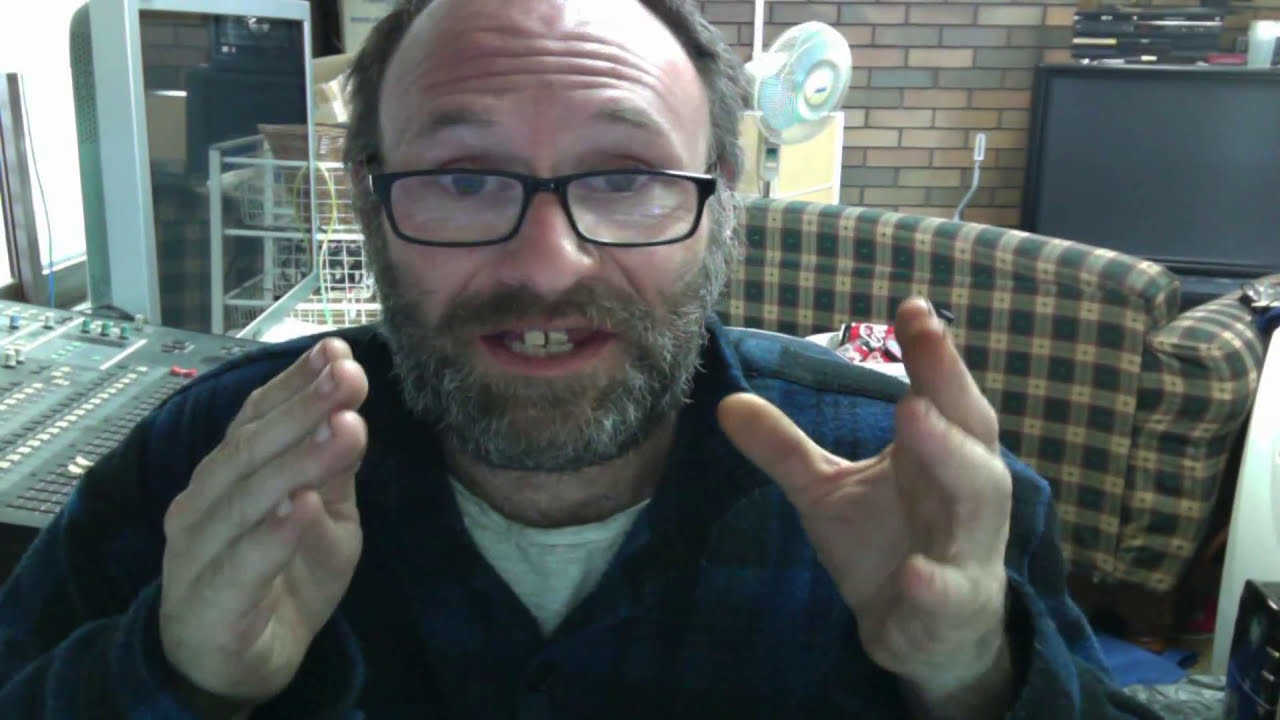In this horizontal rectangular image, a middle-aged Caucasian man is speaking directly to the camera with his hands raised and out to the sides, emphasizing his speech. He is wearing black-rimmed glasses and has a mainly bald head with light brown hair on the back and sides. His somewhat thick, gray and brown beard frames his open mouth, revealing his top and bottom teeth. He is dressed in a blue and black plaid flannel shirt over a white undershirt. 

The setting appears to be a home studio or living room, suggested by a mix of musical and household items in the background. To the left of the man is a large control panel commonly used for music, characterized by visible fader switches, including two white and one red. To the right, an older-looking green and brown plaid couch is partially visible, along with a TV screen in the upper right corner that's turned off. Behind him, a brick wall extends across the background, accompanied by a window on the left side allowing light to shine through. The overall color palette includes shades of brown, gray, blue, white, and light brown.